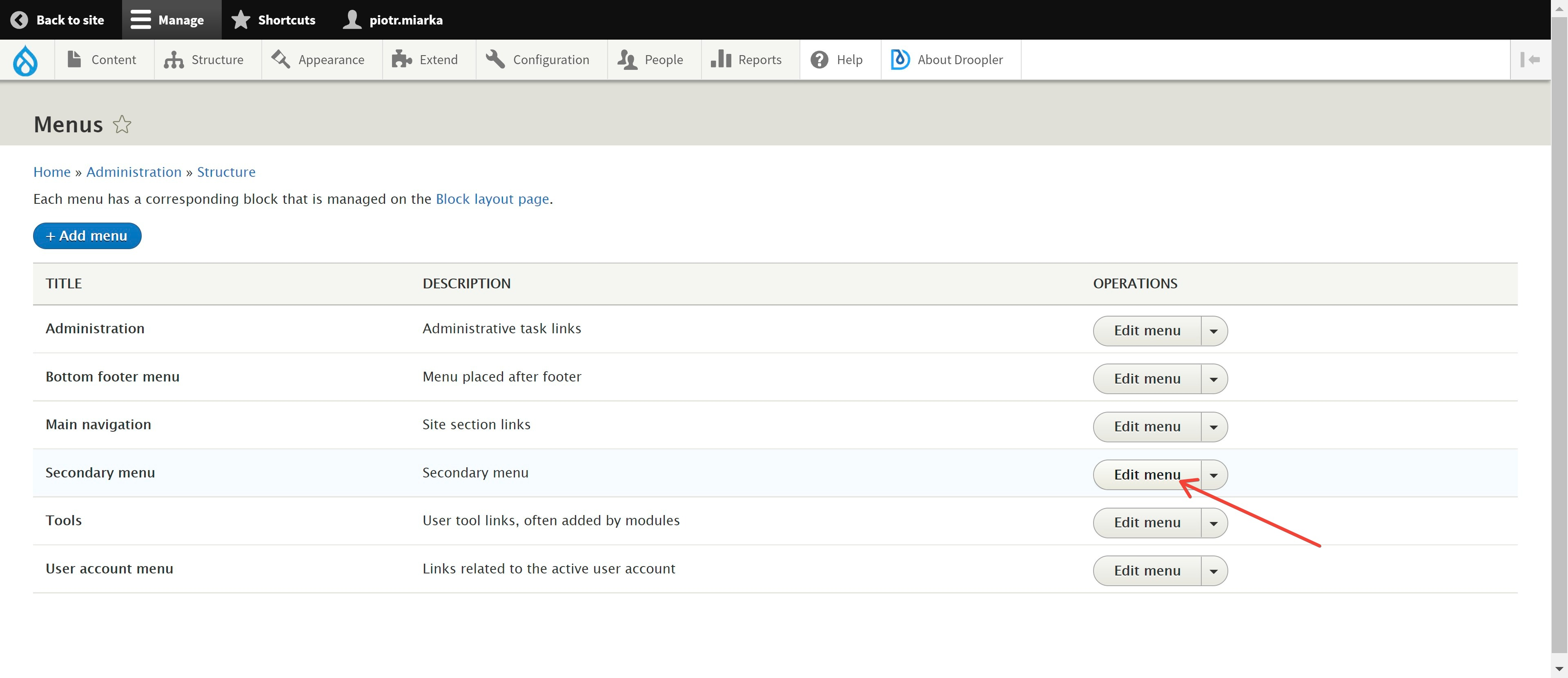This image captures a screenshot of a website's administrator dashboard. At the top of the dashboard, a grey navigational menu is displayed, featuring options such as "Content," "Structure," "Appearance," "Expand," "Configuration," "People," "Reports," "Help," and "About Developer." Below this menu, breadcrumbs indicate the current location within the dashboard, showing "Home > Administration > Structure."

The main section of the dashboard is divided into three columns. The left column lists various menu options such as "Administration," "Bottom Footer Menu," "Main Navigation," "Secondary Menu," "Tools," and "User Account Menu." The central column provides descriptions for these menu items. The right column, labeled "Operations," contains light grey, rounded rectangle buttons labeled "Edit Menu." A prominent red arrow is drawn, specifically pointing to the "Edit Menu" button that is the third from the bottom, drawing attention to this specific option. 

The overall background of the dashboard is white, providing a clean and organized interface for the administrator to manage the website's content and structure efficiently.